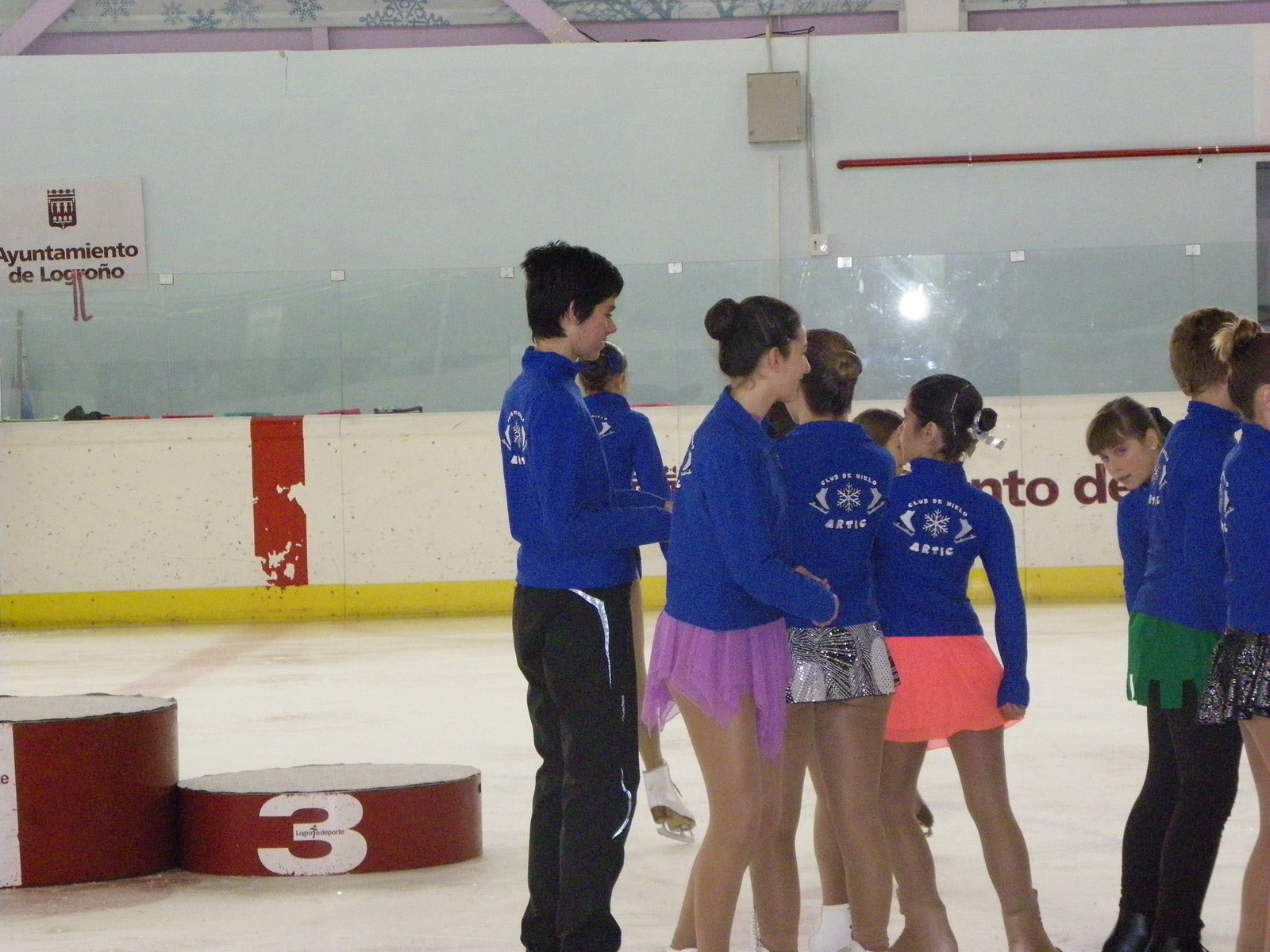This image captures a group of teenage ice skaters, possibly at the end of a competition. The skaters, primarily girls with a couple of boys, are gathered on the ice. They are dressed in matching blue fleece jackets with a logo on the back that includes a snowflake, two ice skates, and the word "Arctic." The girls are wearing skirts in various colors: purple, gray and white, peach, and green, while two boys are in black pants. In the background to the left, you can see the platforms for competition winners, showing the numbers for first and third place. A white solid fence with a red stripe runs along the side, and a sign reads "Ayuntamiento de Logroño," indicating a Spanish-speaking location. The skaters appear happy, with smiles on their faces, suggesting a celebratory moment.